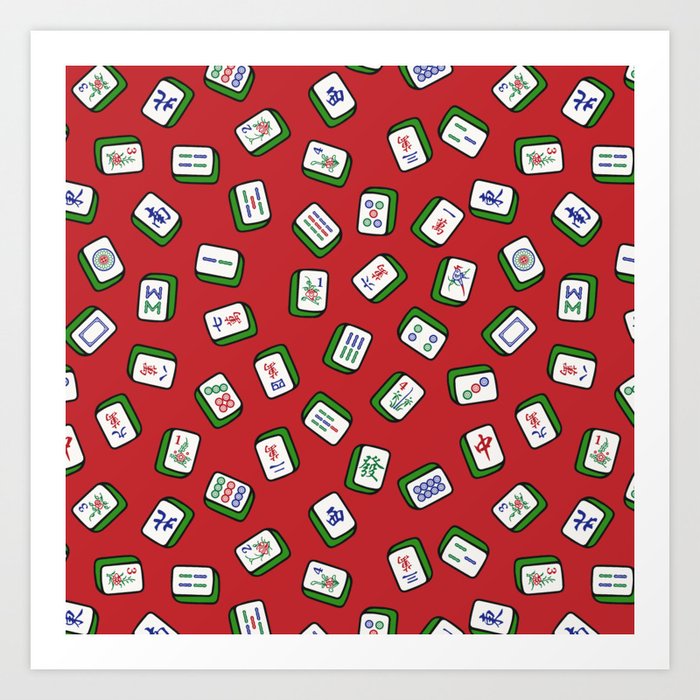This detailed drawing features a vibrant red background overlaid with an assortment of mahjong tiles, numbering between 50 to 100. Each mahjong tile prominently displays a white front adorned with various symbols, including circles, slants, numbers, flowers, and Chinese characters, while the sides and backs are a consistent green. The tiles are meticulously scattered across the red backdrop, showcasing intricate designs in blue, green, and red ink. Specific tiles include one with an upside-down elm, another with 3 circles indicating the number 3, tiles with 2 and 3 slants representing numbers 2 and 3 respectively, and one with 10 circles signifying the number 10, among others. This artistic, cartoonish illustration captures the essence of mahjong, highlighting the diversity and vividness of its tiles.